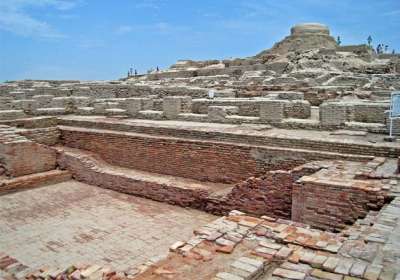The photograph captures an expansive and detailed outdoor scene, taken during the daytime, showcasing ancient architectural ruins set against a partially cloudy blue sky. The ruins, seemingly a demolished fortress or castle, are constructed from a blend of brown, red, and gray stones and bricks, indicative of a historic desert settlement. 

The foreground features broken bricks and scattered debris, suggesting the remnants of a once-grand structure. Central to the image is a hollow section with steps, hinting at former pathways or entrances. Flanking this central area, various levels and walls display intricate brickwork, with reddish-orange hues dominating the lower sections and light gray stones marking the upper terraces.

In the distance, a towering structure resembling a dome-topped tower rises prominently, serving as a focal point that draws the eye upwards and towards the right. The setting is populated with figures that appear to be people, and there is sparse vegetation dotted around, adding life to the historical tableau. The presence of a single cloud in the top left corner adds a touch of atmosphere to the clear, daytime sky, rounding out this vivid and textured snapshot of a bygone era.